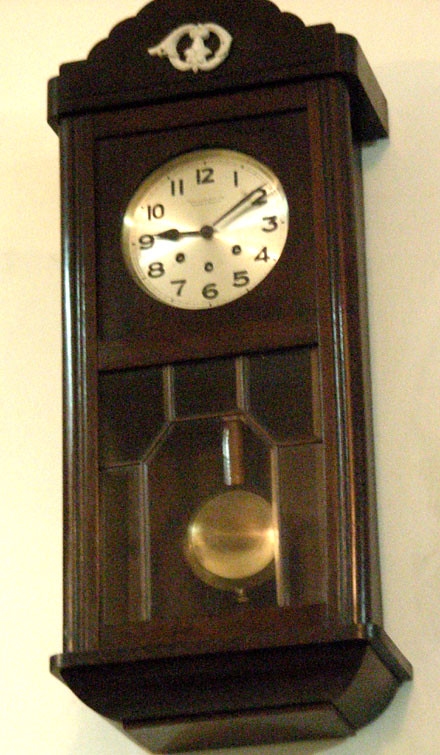The image features a beautifully carved vintage wall clock with a pendulum. The clock boasts a classic, old-style design. The clock face is shiny and displays all twelve numerals clearly. Atop the clock face, there's a circular white design featuring a star with a crown in the center. The pendulum swings gracefully beneath, visible through a glass panel adorned with an intricate pattern, adding to the clock's ornate charm.